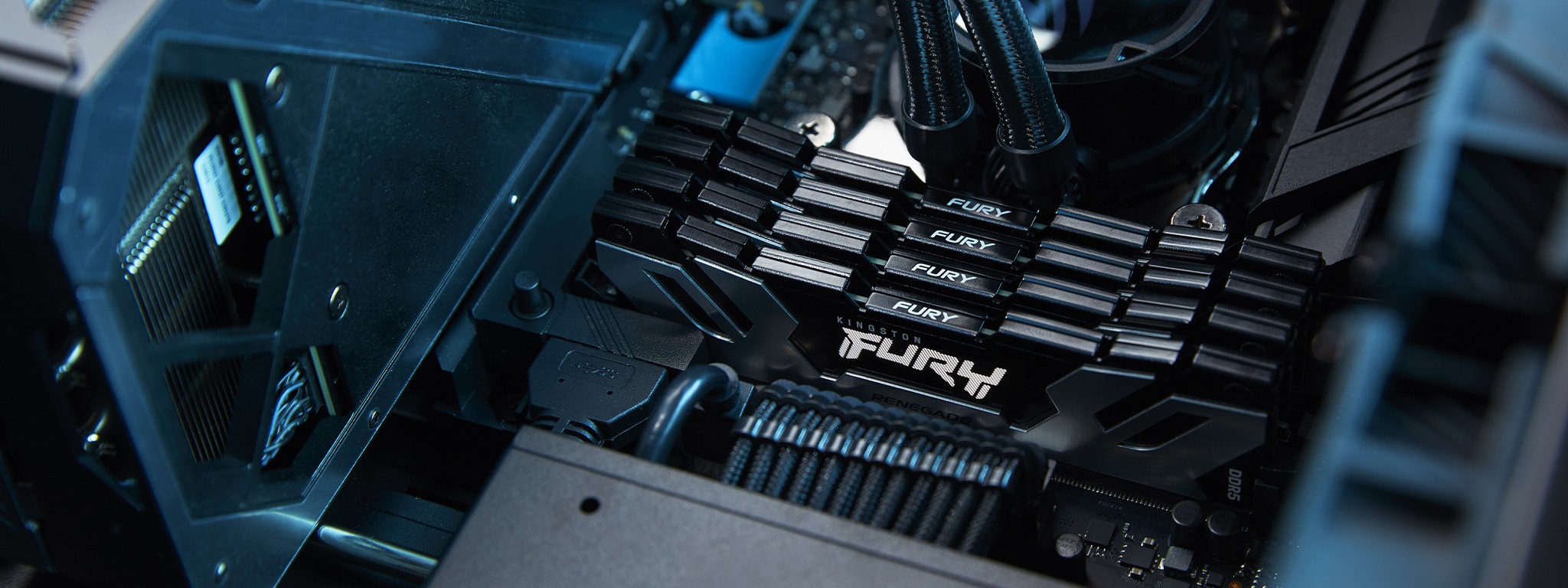The image showcases the interior of a custom-built computer, with a focus on four stacked black RAM sticks labeled "Fury" in white text. The RAM sticks are compact and aligned in a metal bracket, slightly smaller than typical. Extending from the bottom of the RAM sticks are cables, which might be power chords, and from the top, two cloth-like wires are visible. Surrounding the RAM, the case also features reflective metallic gray surfaces, a CPU water cooling system with tubes, and a computer fan positioned above the components. The left side of the image includes a plexiglass area, contrasting with a blurry blue section on the right, highlighted by a detailed, high-quality zoom-in that emphasizes the precision of the electronic setup.